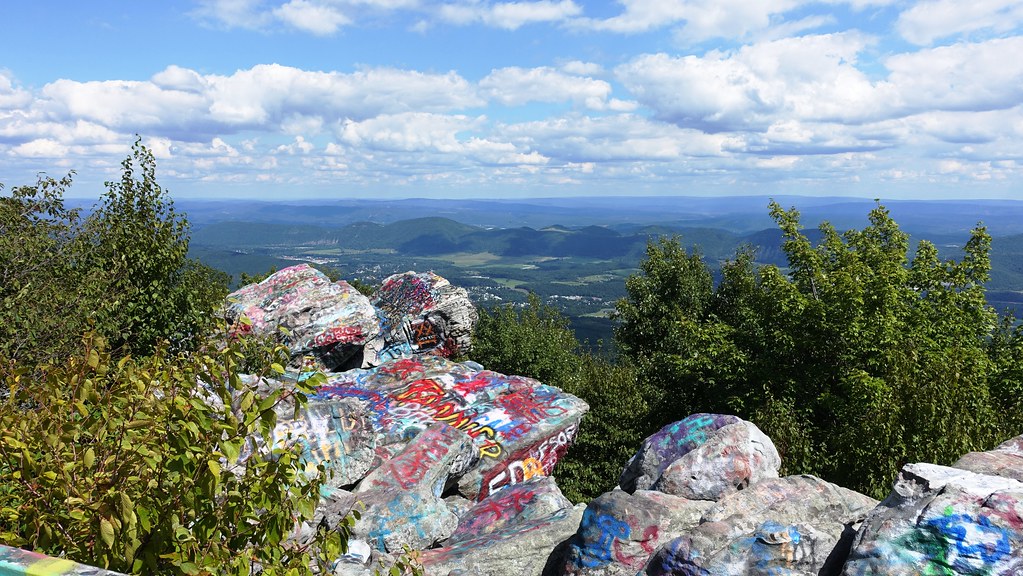This professionally captured photograph presents a stunning high vantage view from a rocky mountain or large hill. The jagged gray and white stones in the foreground are densely covered with colorful graffiti in hues of red, white, blue, purple, orange, and yellow, although the words are indiscernible. Tall trees with green to yellowish-green leaves flank the area, adding a touch of nature's grandeur amid the artistically defaced rocks. The scenic expanse stretches far into the distance, revealing a vast landscape of verdant, blue, gray, and purple mountains, which appear diminutive and far off on the horizon. A light blue sky adorned with fluffy, painted-like clouds, both white and gray, frames the upper portion of the image, completing this serene yet intriguing tableau. Notably absent are any people or animals, allowing the rugged, graffiti-imbued rock formations and distant cityscape and mountains to claim the viewer's full attention.